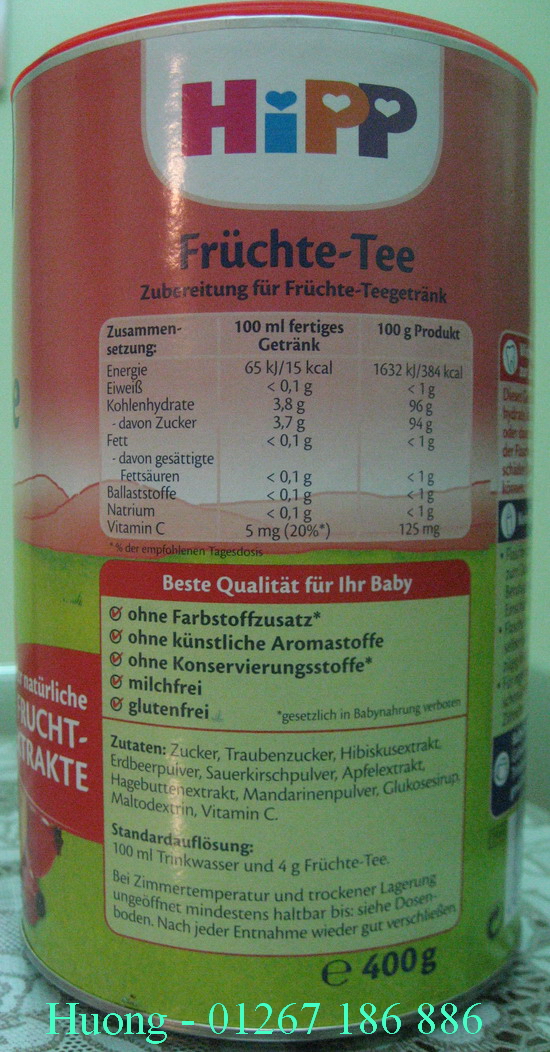This indoor color photograph captures the backside of a food container, potentially baby food, labelled entirely in a non-English language, possibly German. The container, which could be an aluminum or large glass jar, shows a two-tone label: light red on the upper half and light green on the lower half. At the top of the label, there is an oval logo with the brand name "HIPP," featuring white hearts within the letters "P" and a blue heart above the "I." Directly below, black text in French is visible, followed by a light pink rectangle listing nutritional facts in about six or seven lines. In the green portion, more text can be seen, assumed to be in German, along with a light green overlay of text reading "HUONG-01267186886." The bottom of the label also displays "400G" in black text. The photograph includes a glimpse of the gray, floral-patterned placemat on which the container rests.